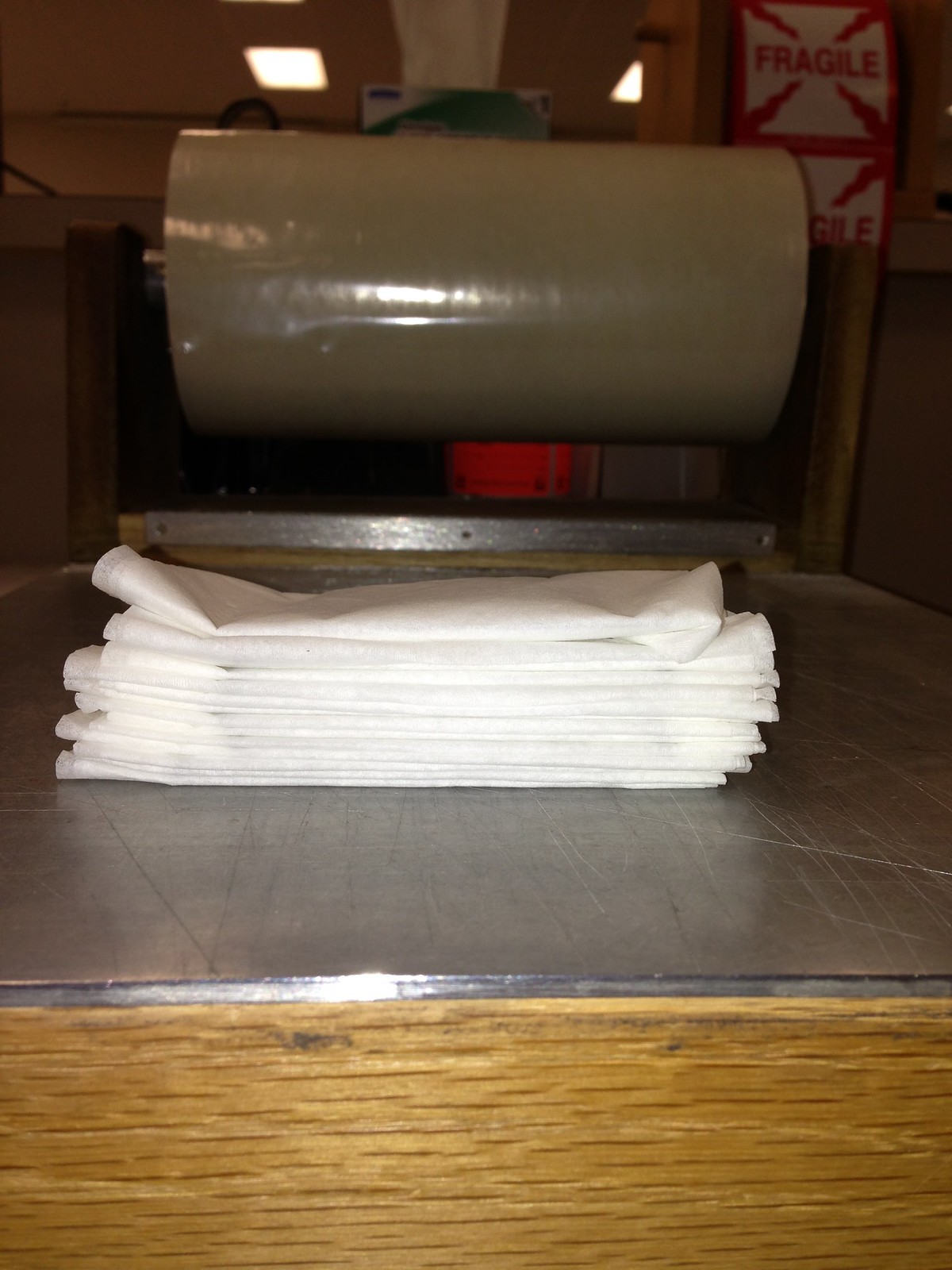The image depicts a close-up scene inside a warehouse, showcasing what appears to be a mailing station. At the very front, there is a light oakwood table with a layer of metallic countertop that is heavily scratched, suggesting frequent usage. Resting on this surface is a neatly stacked pile of white napkins or similar folded sheets. In the background, there is another metallic surface topped with a roll of packing tape, which is thick and shiny, commonly used for sealing packages. Positioned to the top right corner, there is a distinct label that reads 'Fragile' in red text within a white square, adorned with red lightning symbols at each corner. This detailed setup indicates a well-used station designed for preparing and wrapping items for shipping.